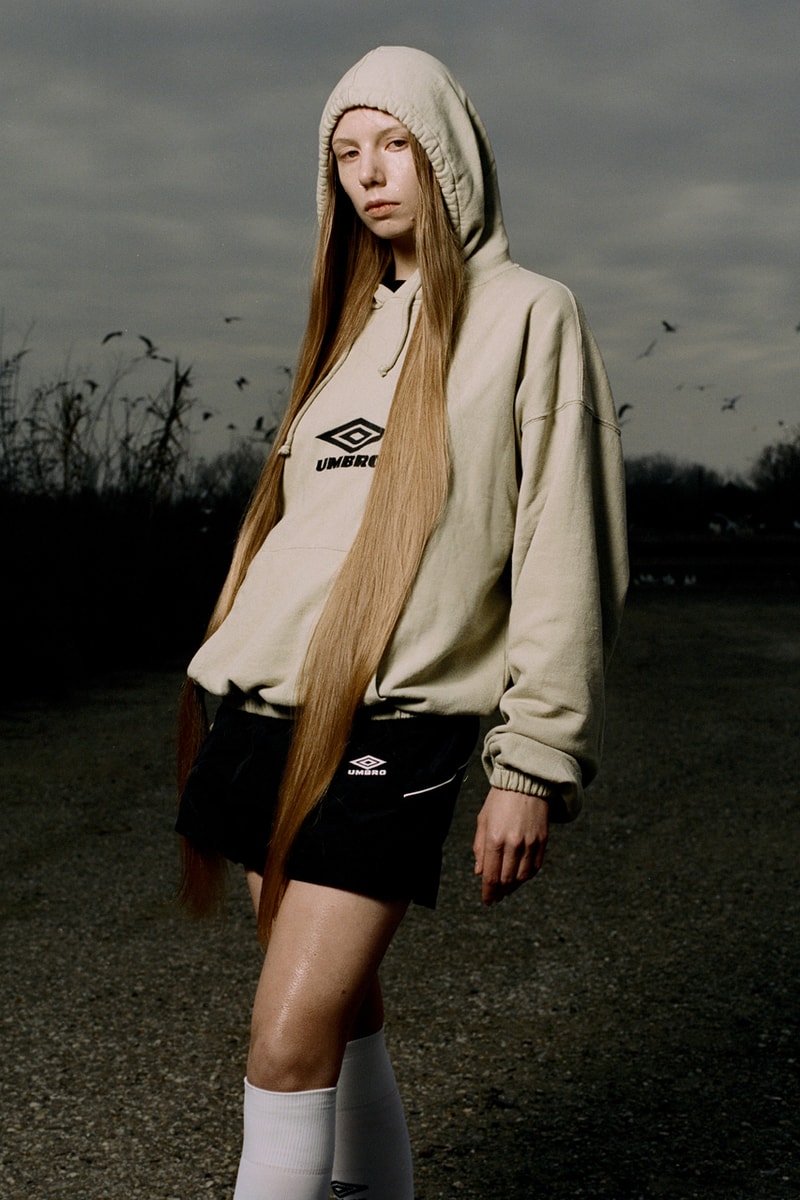The image captures a young adolescent girl standing outdoors on a gloomy day. She has pale white skin with a slight shininess around her kneecaps and very long, golden-brown hair cascading from her hooded head down to her knees. She wears an oversized beige hoodie with the Umbro logo and name printed in black on her chest, the hood covering her head but allowing her hair to flow out on either side. Her black shorts, also by Umbro, feature a diagonal white stripe and the brand's logo near the top. She stands confidently with her legs crossed, her left arm visible while the right remains hidden. Tall, green weeds and a darkened, charcoal ground form the backdrop, contrasting with the cloudy, dim sky above, giving the scene a moody, almost stormy atmosphere. White knee-high socks complete her outfit. In the sky, birds are discernible near her right shoulder, seemingly flying away. The photograph appears to have been taken at twilight, capturing the serene yet atmospheric moment in striking detail.